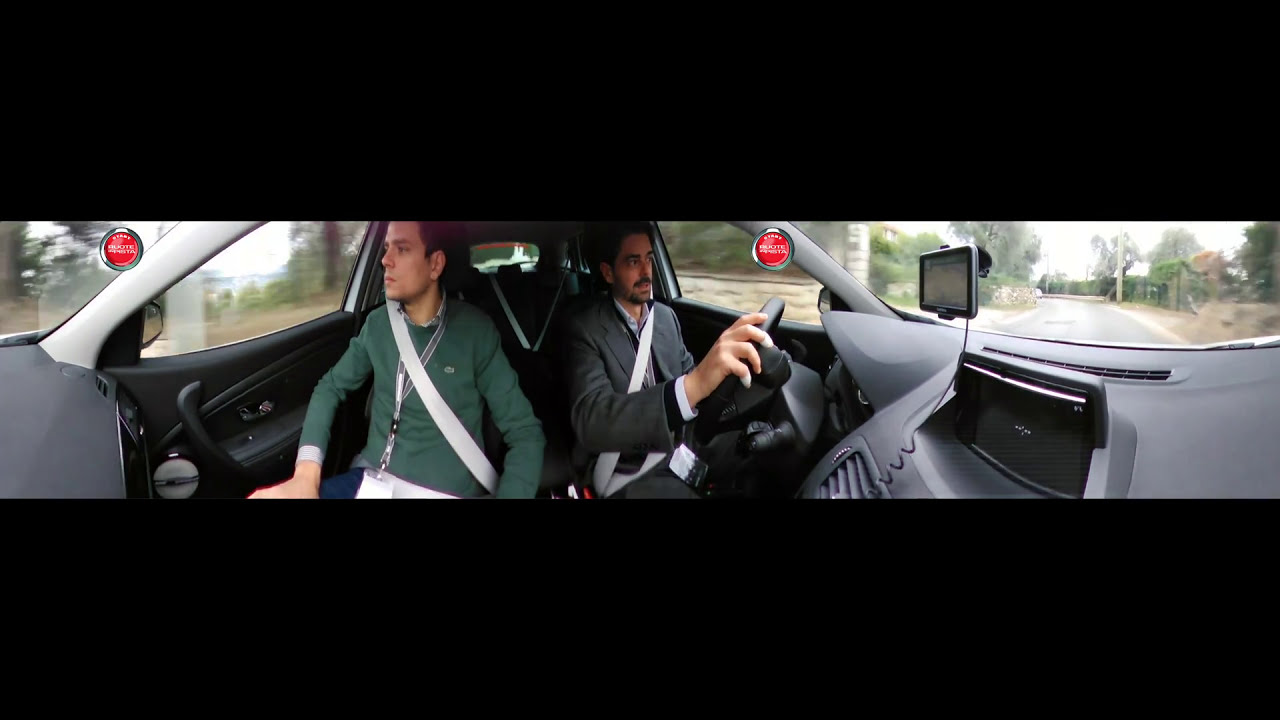This detailed photograph captures the interior of a modern, dark silver car. The centerpiece of this image is two men: the driver and the passenger. The driver, clad in a gray business suit over a white shirt with black cuffs, has a short mustache and beard with black hair. His right hand firmly grips the black steering wheel, and his seatbelt is securely fastened. Notably, he does not wear a tie. Mounted on the dashboard is a GPS device or a dash cam.

The passenger, likely in his late 20s to early 30s, appears Caucasian with short brown hair. He wears a green long-sleeve sweatshirt, adorned with an alligator logo, over a blue collared shirt, and a lanyard with an employee card drapes around his neck. He too has his seatbelt fastened and gazes out the window. 

The car's dashboard features a navigation system and a touchscreen. Through the windshield, a single-lane road unfurls, bordered by trees and illuminated by the midday sky. The scene is framed by a subtle black border, further focusing attention on the two central figures in the car. The primary colors in the image include shades of black, gray, green, blue, red, tan, and silver, suggesting a lively yet composed setting.